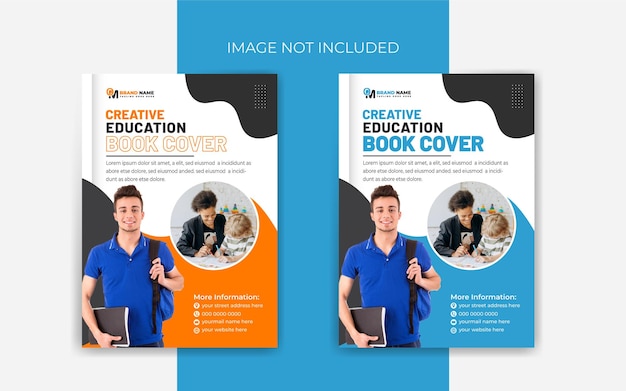The image features two textbook covers set against a background of three blue bands of varying shades. The left cover showcases a predominantly orange, white, black, and dark gray color scheme, while the right cover mirrors this design but with blue replacing the orange. Both covers prominently display the title "Creative Education Book Cover" at the top, along with a smaller text below that changes based on context. 

Each book cover includes identical photographs: a young man in a blue shirt, holding a black notebook in his right hand with a backpack slung over his left shoulder, and an inset circular photo of a woman teaching a small child. The bottom right corner of each cover also features some additional smaller text. The overall design is consistent between the two covers, with the primary difference being the shift in color scheme from orange to blue.